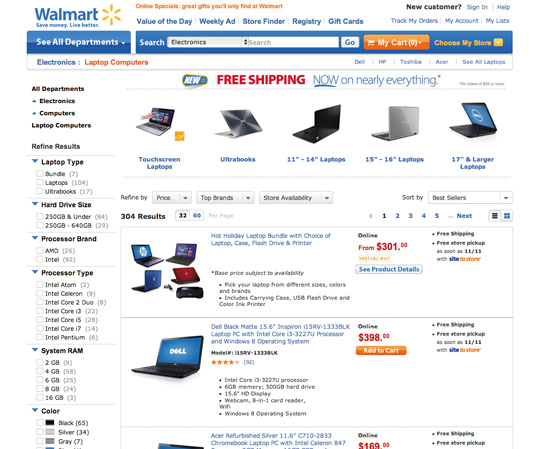Screenshot of Walmart Website Interface:
The image is a detailed screenshot from the Walmart website, with the iconic Walmart logo prominently displayed in the upper left corner. The logo features "Walmart" in blue lettering accompanied by a yellow asterisk-like design to the right. 

The top navigation bar includes several clickable options: "Value of the Day," "Weekly Ad," "Store Finder," "Registry," and "Gift Cards." In the upper right corner, there is text in black font posing the question "New customer?" next to blue-font buttons for "Sign In" and "Help." Beneath these, a rectangular white search bar stands ready for product queries. To the right of the search bar, an orange rectangular button with white text reads "My Cart," currently showing zero items, and is accompanied by a shopping cart icon.

The primary section of the screenshot reveals that the user has searched for laptops. Displayed products include various laptop brands such as Dell and Hewlett-Packard. At the top of the page, categories for different types of laptops are listed, such as "Touchscreen Laptops," "Ultrabooks," "11-inch to 14-inch," "15-inch to 16-inch," and "17-inch and larger." The left side of the page features sorting options by brand, allowing users to filter through the laptop selection more efficiently.